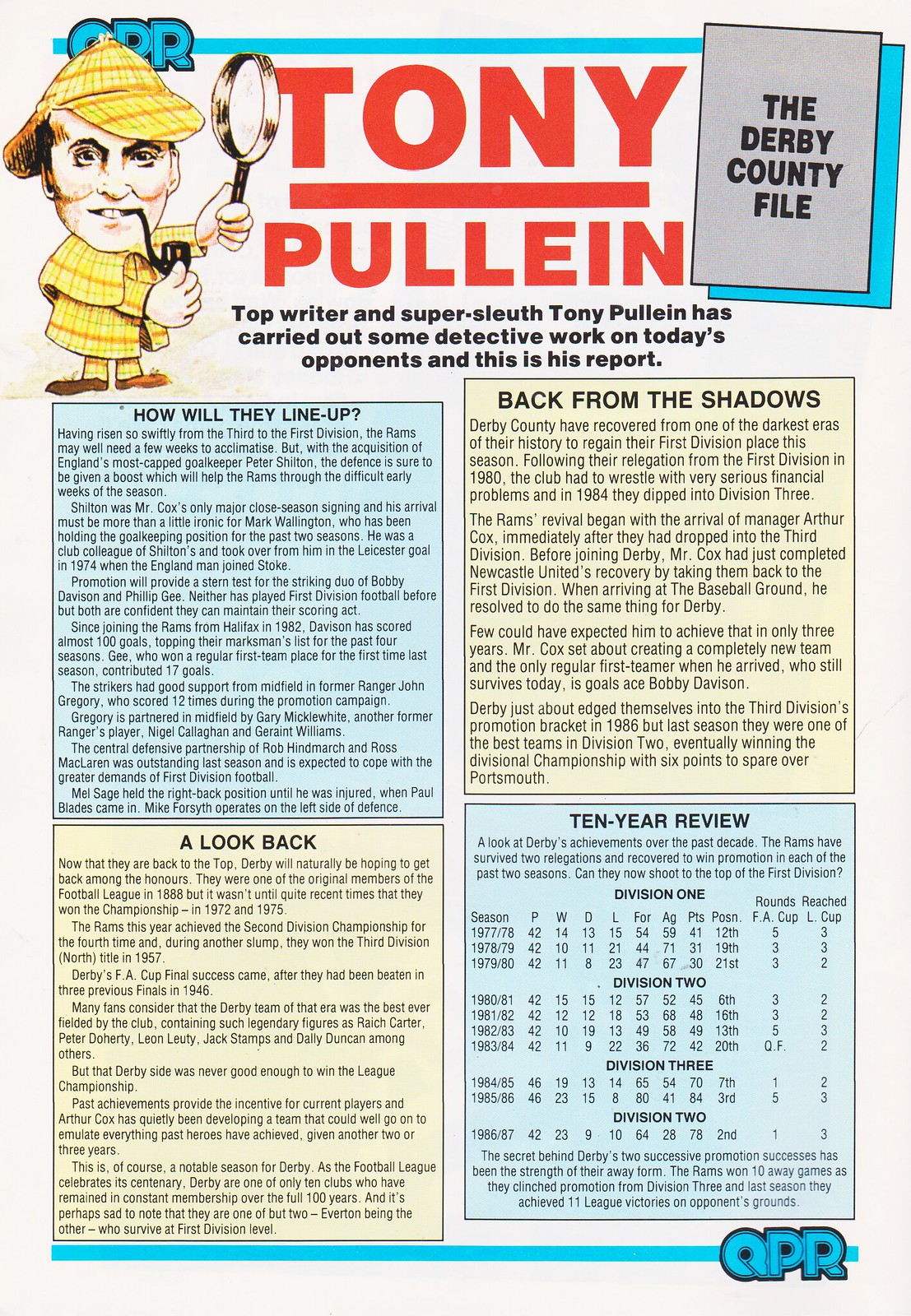This image resembles a lively and vibrant magazine page, primarily discussing English football, specifically focusing on Derby County and their opponents. At the top, in bold red text, it announces "Tony Pullian," a "top writer and super sleuth" who has done investigative work on today's opposing team. A playful cartoon character, dressed as a detective with a yellow outfit, magnifying glass in hand, and a pipe in his mouth, is situated to the left of this text. Below, the page is divided into four colorful quadrants: 

- The top left quadrant features a blue background with black text under the heading "How will they line up," likely analyzing team formations.
- The top right quadrant, with a yellow background and black text, is titled "Back from the shadows," perhaps discussing returning players or team dynamics.
- The bottom left quadrant, also on a yellow background, is headed "A look back," focusing on historical insights or past performances.
- The bottom right quadrant presents "10-year review" on a blue background, showcasing various charts and statistics detailing divisional facts over the last decade.

The detailed captions and varied content suggest a comprehensive sports-themed article designed to engage readers with its colorful layout and diverse information.